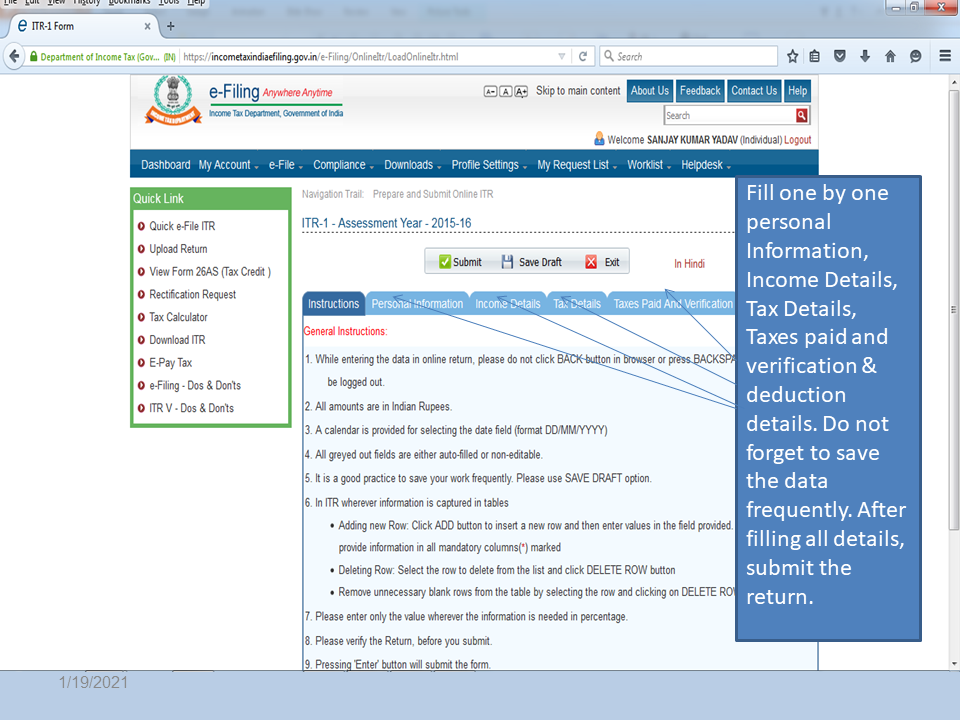The image depicts a web browser interface with a gray border at the top. The browser tab displays an unreadable name, alongside a URL in the address bar. Below the address bar, there's a prominent box with the text "E-filing Anywhere Anytime" and an accompanying logo featuring a red ribbon. On the right side of this box, a link reads "Skip to main content."

The interface includes several buttons: "About Us," "Feedback," "Contact Us," and "Help." Beneath these buttons, a search bar is visible. Directly below the search bar, a dark blue colored menu bar offers a variety of options: "Dashboard," "My Account," "E-file," "Compliance," "Download," "Profile Settings," "My Request List," "Work List," and "Help Desk."

Lower in the interface, there is a green box labeled "Quick Links" containing approximately ten different navigation options.